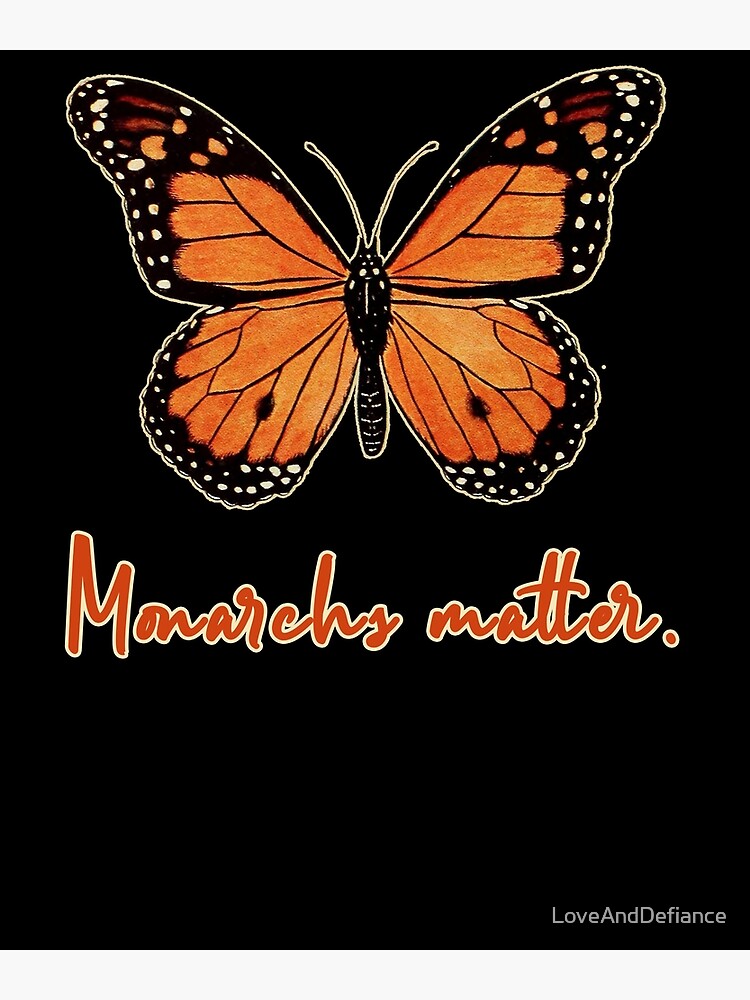The image features a large rectangle with a solid black background. Centrally positioned towards the top is an artistic drawing of a monarch butterfly. The butterfly, with its black body and two long antennae, has four distinct wings. The wings are primarily orange near the body, transitioning to black around the outer edges and adorned with white dots. Additionally, each lower wing has two black spots. Below this detailed illustration, the words "Monarchs Matter" are written in an orange script-style font with white outlining. At the bottom right corner of the image, the phrase "Love and Defiance" is inscribed in white text, adding an extra layer of emphasis to the overall design.